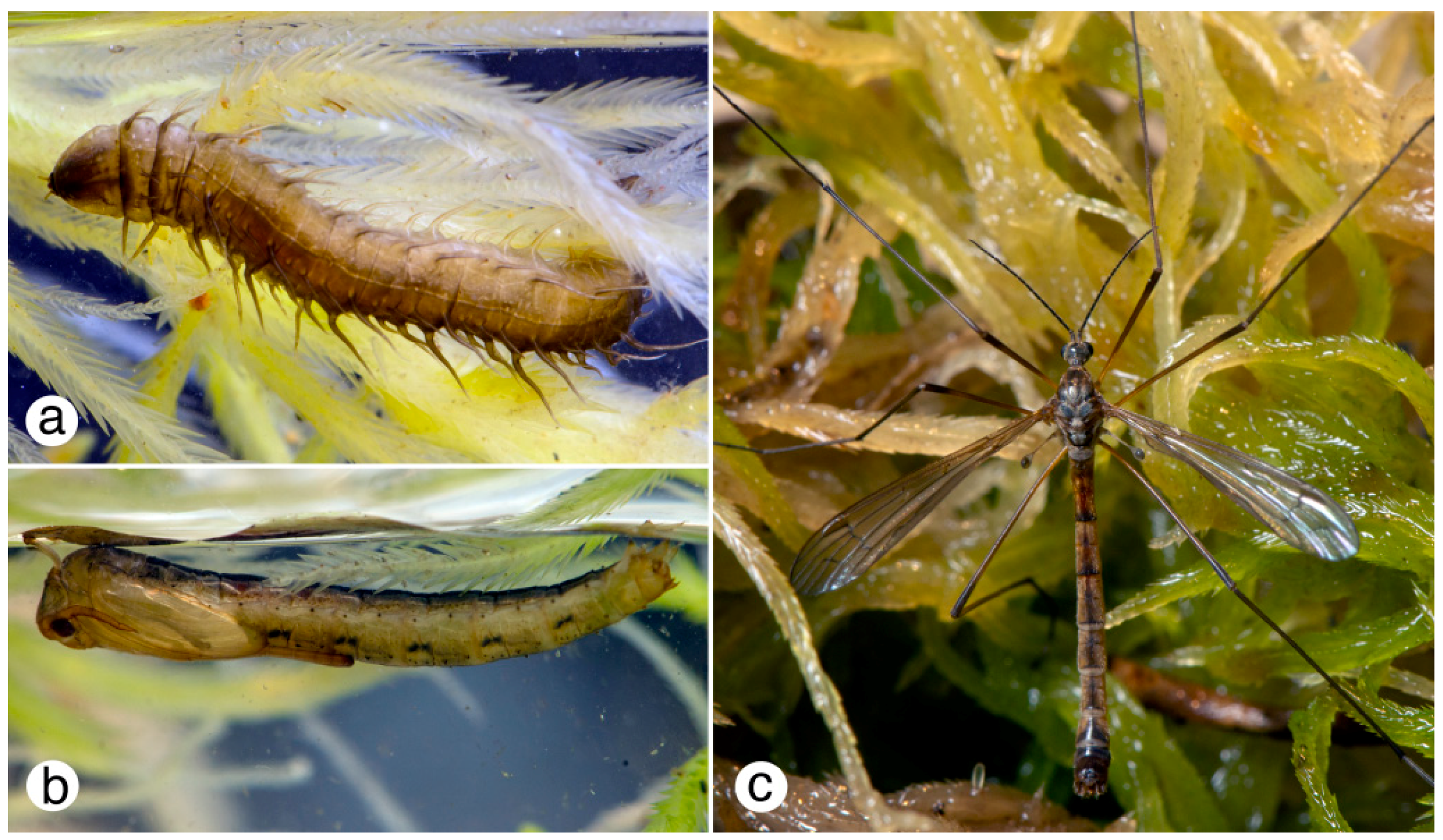This composite image serves as a diagram depicting the life cycle of an insect that resembles a dragonfly or mosquito eater, labeled with three photographs A, B, and C. On the left side, the upper photograph labeled A features a light brown larva, possibly a millipede or centipede-like creature, nestled among greenish-yellow leaves. Below it, photograph B shows another stage of the insect, likely a larva or nymph, appearing to hang upside-down on similar greenish hue leaves. Both A and B share a setting with natural elements in the background, possibly aquatic or wet. Dominating the right half of the image, photograph C showcases the mature insect, characterized by a long, slender, brownish-beige body with spindly, near-translucent wings and three sets of elongated legs. The head, slightly thicker with prominent features like beady eyes and antennae, is set against a backdrop of verdant, possibly wet, leaves, contributing to the habitat's consistent greenish-yellow theme.